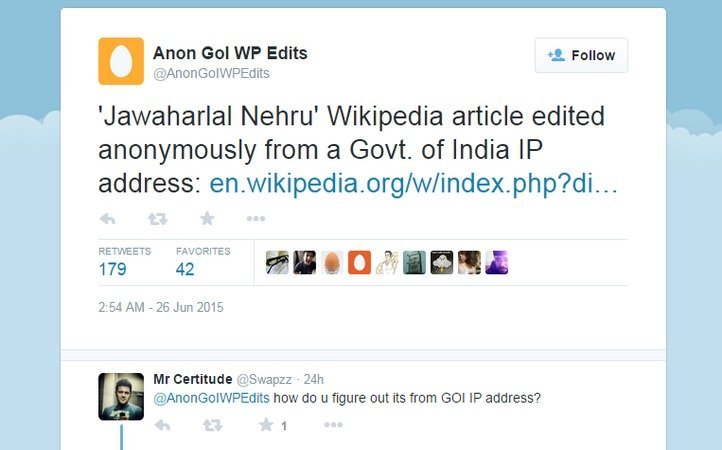The image is a screenshot featuring a tweet displayed against a white background, adorned with narrow, sky-blue borders on the left and right edges. Central to the image is the content of the tweet from Twitter. 

In the top left-hand corner of the tweet, the profile picture is a simple orange square with a white oval in the center. The tweet is authored by the user "AnanGolWPedits." The accompanying display name appears to be: "JAWAHARLAL Nehru Wikipedia article edited anonymously from a government of India IP address," though the exact pronunciation of the name is not provided.

The tweet includes a hyperlink in blue text, "en.wikipedia.org," indicating the web address of the related Wikipedia page. Below the main content, the tweet has amassed 179 retweets and 42 favorites. The timestamp at the bottom indicates that the tweet was sent at 2:54 AM on June 26, 2015.